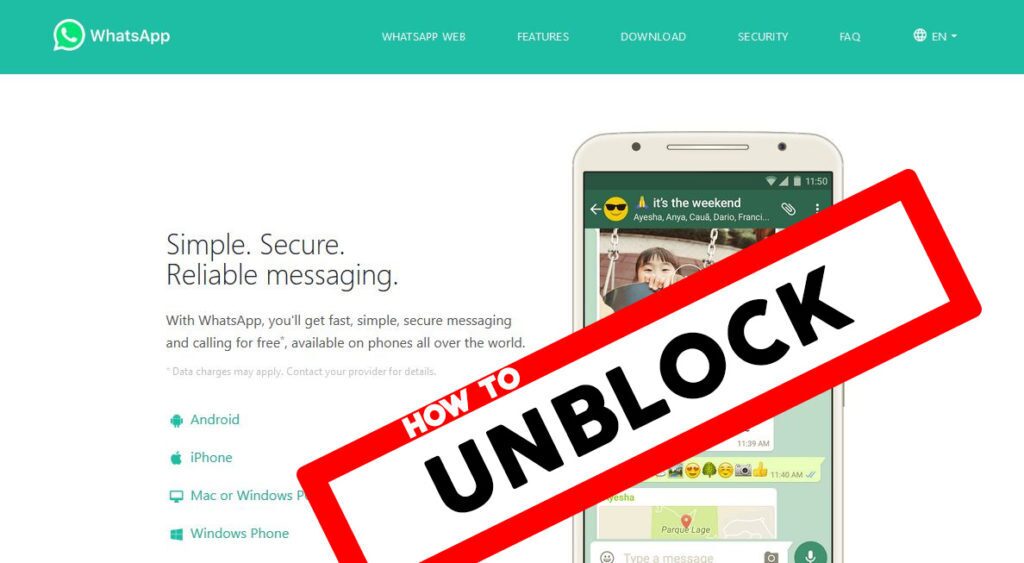This is a caption that somebody gave for an image using their voice. Clean it up and formulate it into a descriptive caption. Make it very detailed.

Original:

This is a web page that has a green header. In the upper left-hand corner, it says, WhatsApp has a green WhatsApp logo. Look to the right, there is a header elements, WhatsApp web features, download, security, FAQ, and a globe and EN. This is all in white text on a green background in the header. If we go down to the body of the page, on the left-hand side of the body, it says simple, secure, reliable messaging with WhatsApp, you'll get fast, simple, secure messaging and calling for free available on phones all over the world. Underneath that, it says Android, iPhone, Mac, or Windows Phone, or Windows PC, I think actually. It's covered by this red box that says how to unblock with a red border, and it says how to in white. Then in the white background, the background is white in the middle of it, and then it has black text in bold. Then this is over a phone that looks like an Android device, and it has a picture of WhatsApp on it. Header is green. It looks like it's in a group chat. It says, it's the weekend, and it has the names of the individuals there, and it has the messages, and that's it.

Cleaned and Detailed Caption:

This web page features a green header with a white WhatsApp logo in the upper left-hand corner. To the right of the logo, the header contains navigation elements, which are displayed in white text: WhatsApp Web, Features, Download, Security, FAQ, a globe icon, and "EN" indicating the English language. 

In the main body of the page, prominently displayed on the left-hand side, there is bold, black text on a white background that reads: "Simple, Secure, Reliable Messaging with WhatsApp." Below this, it continues: "You'll get fast, simple, secure messaging and calling for free, available on phones all over the world." A list of devices – Android, iPhone, Mac, and Windows PC – follows this message, although part of it is obscured by a red box with a red border. Inside the red box, there is white text reading "How to Unblock."

The page also features a visual of an Android phone, displaying a WhatsApp group chat. The chat screen shows a conversation with the message "It's the weekend," along with the names of the participants and their individual messages. The header of the chat is green, maintaining the consistent color theme of the webpage.